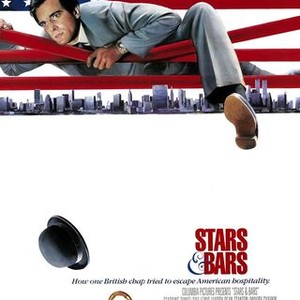The image is an advertisement, likely a movie poster for "Stars and Bars," presented by Columbia Pictures. Dominating the visual appeal is a man with black hair, dressed in a gray suit and dark dress shoes. The man is scaling through what appears to be a red-striped fence that resembles the American flag. His left arm and left leg are draped over one of the red stripes, indicating movement. He wears a watch on his left arm, and his one leg is crossed over the stripe, with his shoe still on.

Above the man, stars occupy the top left corner, while below him lies a distant city skyline, suggesting New York. The bottom half of the image is predominantly white space, save for a black hat positioned upside down at the very bottom center. On the right side of this white space, the title "Stars and Bars" is written in red, capital letters. The tagline underneath reads, "How one British chap tried to escape American hospitality." Small, hard-to-decipher black text follows, likely listing additional details about the film.